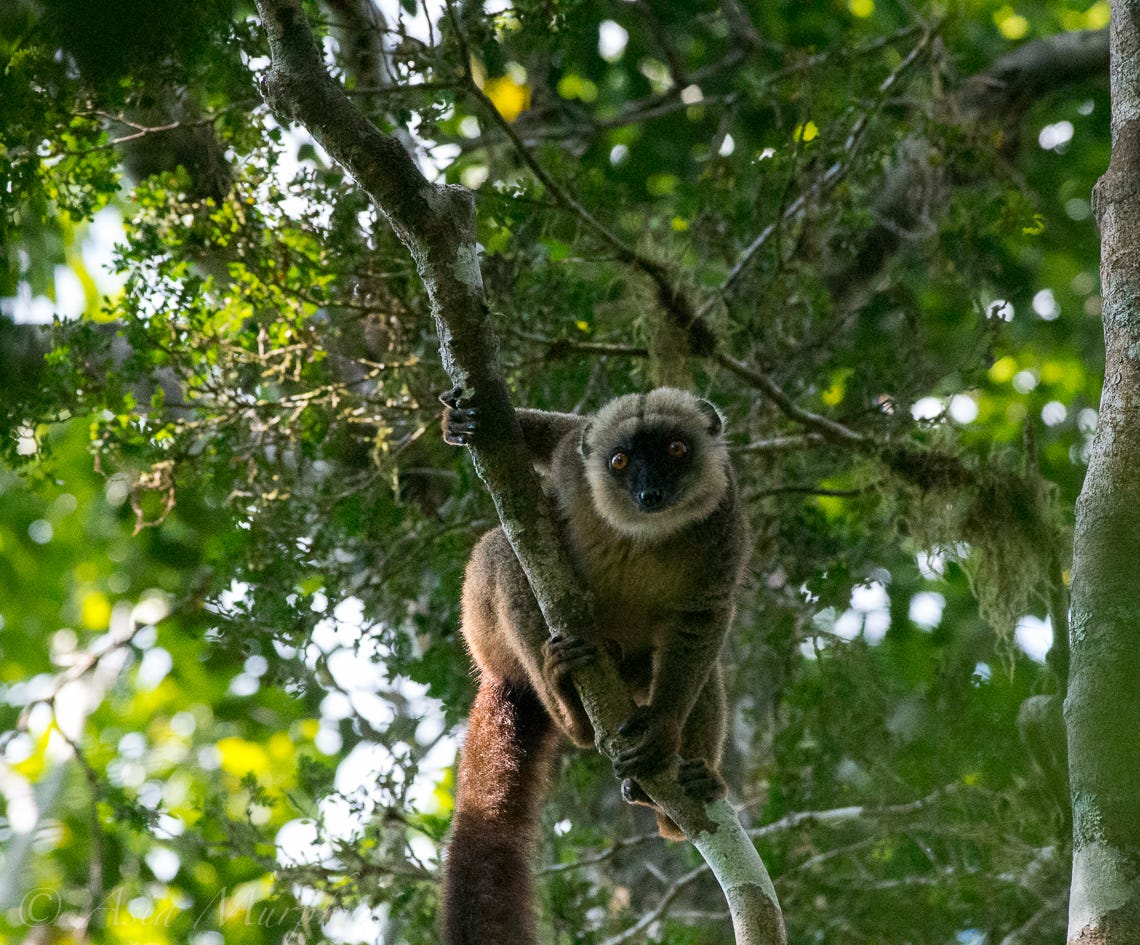This photograph features a lemur perched on a thin, brownish-green tree branch amidst a dense, tree-filled background. The lemur, centered in the image, grips the branch with all four limbs and gazes directly at the camera. It has large brown eyes set against a black face, framed by white, bushy fur. The lemur's body is covered in thick, bushy brown fur, and it has a notably long, bushy tail hanging down. The natural setting includes various tree branches draped with moss and green leaves, creating a vivid, nature-rich backdrop. The photograph is square, and there is a faint copyright text in the bottom left corner, although the name is not clearly discernible against the sky.